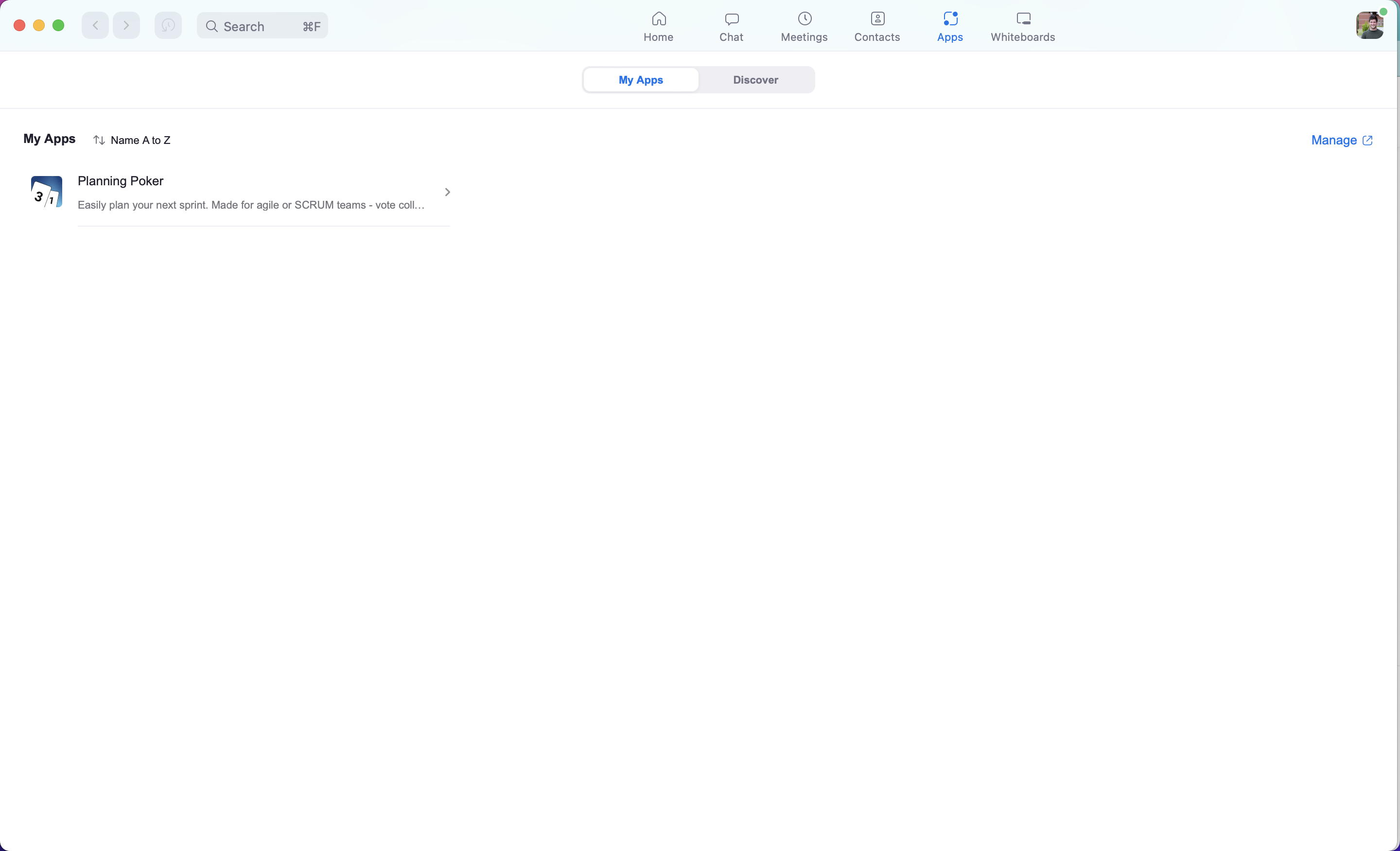A computer screen snapshot displays the active desktop of a software developer, likely used for tracking ongoing projects. The interface features a primarily blank page with minimal information. At the top, a light blue-gray bar extends across the screen. On the upper left corner, it contains three dots in red, yellow, and green, followed by a back arrow, a forward arrow, a reload button, and a search box. 

On the far right side of the top bar, a series of icons is displayed, representing home, chat, meetings, contents, contacts, apps, and whiteboards functions, respectively. Below this top bar, on the left side of the screen, text reads "My Apps: name A to Z.” Accompanied by a blue icon featuring two white squares, labeled with a '3' on the left and a '1' on the right.

The app named "Planning Poker" is highlighted with a description that reads: "Easily plan your next sprint made for agile or scrum teams. Vote COLL..." (cut off on the right side). On the top right of this section, there’s a blue "Manage" button followed by an arrow.

This interface succinctly combines elements for navigating through various apps and tools, focused on agile project management practices.